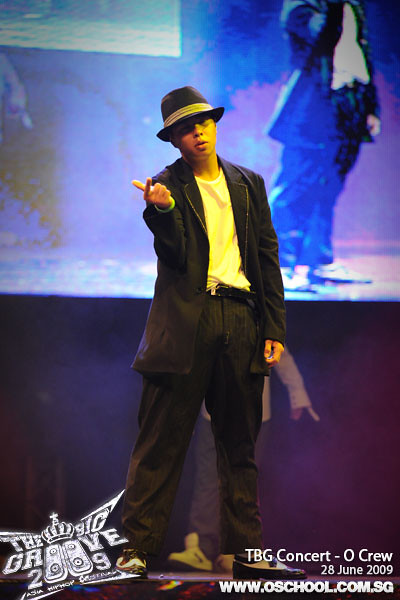A young man with brown skin is performing on stage, dressed in an oversized black dress jacket, slacks, a black dress hat with a brim and a yellow bandana at the base, and a white T-shirt which appears slightly yellow due to light reflection. His black dress shoes complete the ensemble which resembles Michael Jackson's iconic style. The performer stands with his feet shoulder-width apart, his left hand down at his waist, and his right hand raised with his thumb and index finger forming an "L" shape, suggesting he's in the middle of a musical performance. His eyes are closed, seemingly immersed in singing. The top half of the rectangular photograph, taken indoors, shows a projection of the live event, creating an LED backdrop effect behind the performer. The dark background contrasts with the blue backdrop at the top. The photograph also includes textual elements: at the lower right-hand corner, it reads "TBG Concert Oak Crew, 28 June 2009, www.oschool.com.sg" and at the lower left-hand corner, there is a logo featuring a crown with the inscription "The Big Groove, 2009."